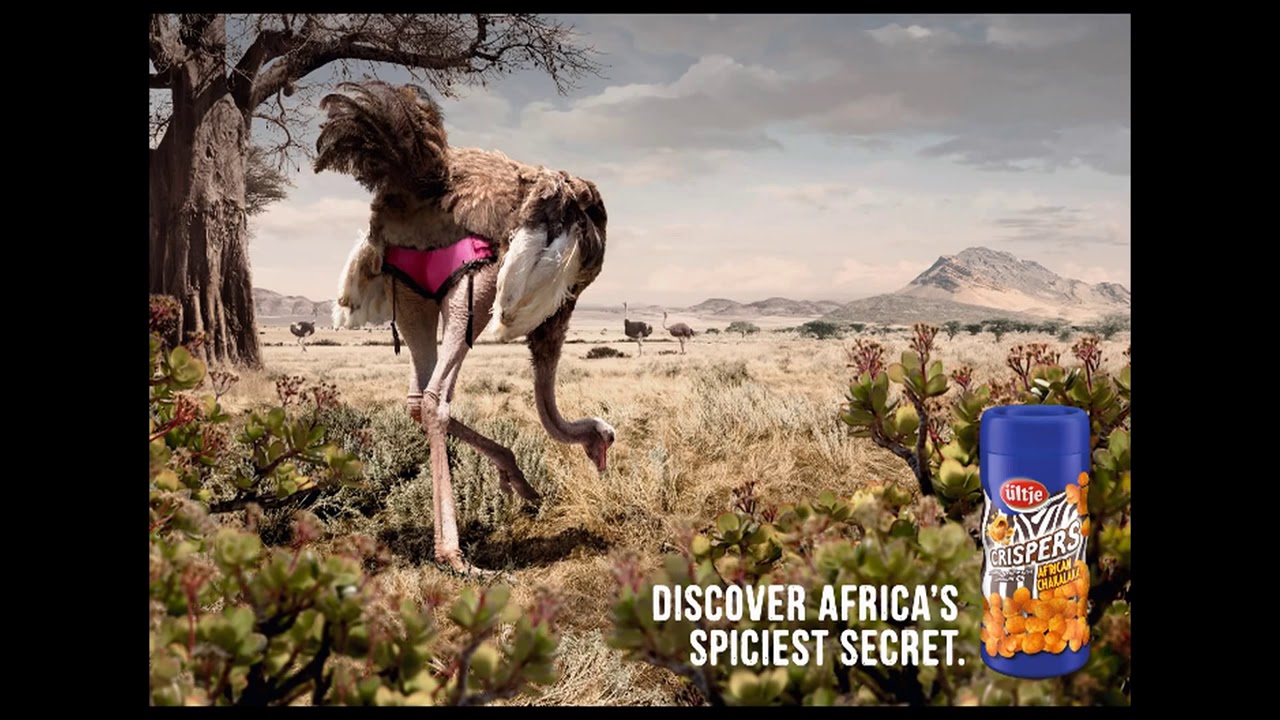The whimsical advertising poster captures an entertaining and unusual scene set in a savanna-like landscape. The background features a vast sky with wispy clouds and distant mountains – smaller peaks on the left and a larger one on the right – shrouded in a gray haze. The foreground portrays a dry scrubland populated by green bushes, sparse brown straw-like patches, and a prominent tree with tiny leaves situated on the left side. Central to the image is an ostrich, humorously adorned in pink lacy panties with black trim, bending down to peck at the ground. The surrounding area teems with details like scrub brush and pinkish flowers. In the bottom right corner, white text reads "Discover Africa's Spiciest Secret." Adjacent to this, a blue-topped container labeled “CRISPRS” displays images of coated nuts or corn pieces, with a red oval about a third way down, and some harder-to-read yellow text beneath it, possibly adding to the mischievous nature of the advertisement. The image blends humor and quirkiness, using the odd juxtaposition of the ostrich and the intimate apparel to craft a memorable ad, likely aimed at evoking laughter and curiosity among viewers.